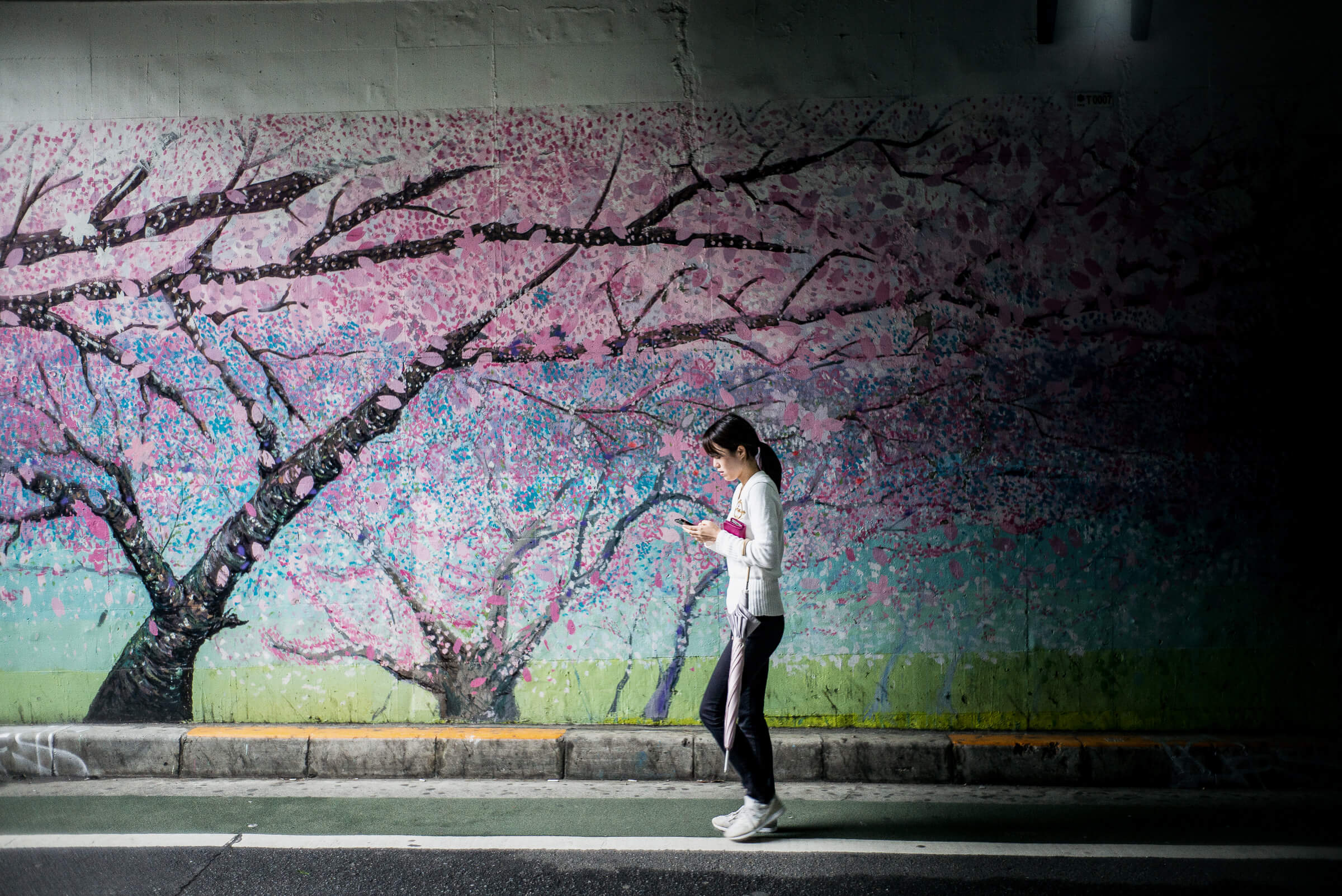A watercolor painting captures a serene spring scene with a young woman engrossed in her phone, walking along a sidewalk. She has dark hair tied in a ponytail, and she dons a long white shirt, black pants, and white shoes. A notable detail is her purple purse, which she carries possibly as a wallet. The walkway she's on is adjacent to a bike lane marked by green paint and white lines, bordered by black asphalt. Nearby, a concrete curb features patches of yellow at the top. 

In the background, a large mural adorns a white stone or brick wall, depicting cherry trees in full bloom with pink and white blossoms. The mural also shows dark branches and green grass at the bottom, with hints of a blue sky peeking midway. The woman seems oblivious to her picturesque surroundings, captured in the act of walking and looking at her phone, possibly holding a white umbrella.